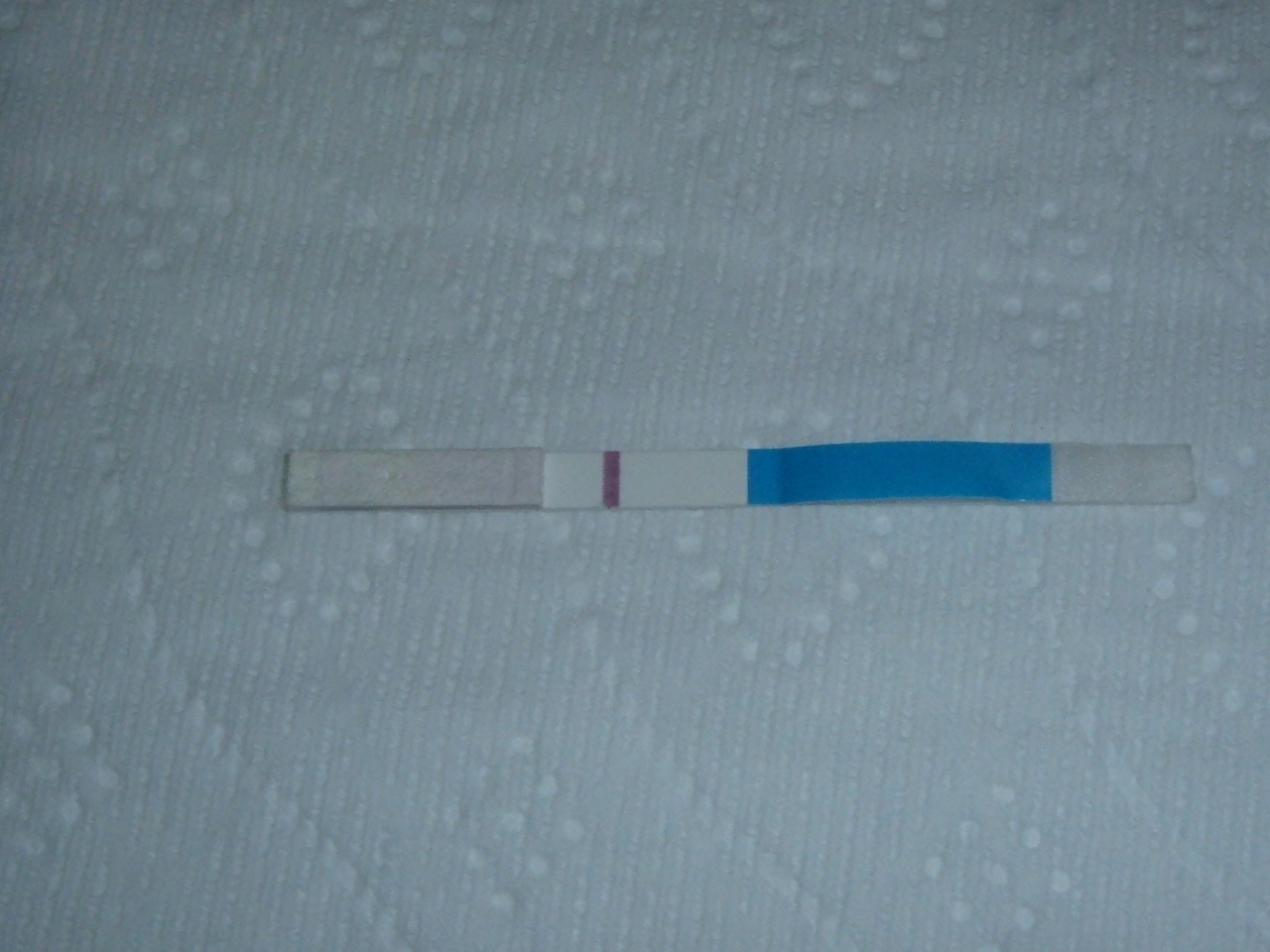The image depicts a close-up of a test strip placed on a piece of patterned toilet paper, identifiable by its diamond-shaped indentations. The test strip is reminiscent of those used in pregnancy or COVID testing, where multiple lines indicate a positive result. However, in this image, only a single line is visible, suggesting a negative outcome. The strip features a clear, whitish section on the left, likely the area where the specimen is applied, and a longer blue section on the right. The intricate details of both the test strip and the toilet paper pattern are prominently highlighted in the zoomed-in shot.